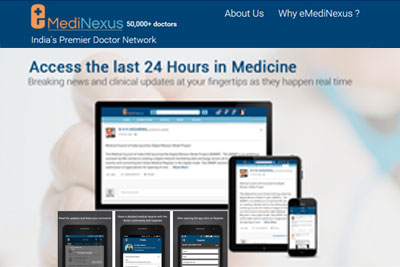A screenshot from the MediNexus website, which is recognized as India's premier doctor network boasting over 50,000 doctors, showcases its user interface on various devices. The top right corner of the screen features clickable buttons labeled 'About Us' and 'YE MediNexus.' The screenshot displays multiple devices, including a horizontal tablet, a vertical tablet, and a cell phone, all actively interacting with the site. Various images and screenshots illustrate the website's features, highlighting sections where users can access the latest 24-hour updates in medicine, breaking news, and real-time clinical updates. The top of the screen is marked by a dark blue text bar with the MediNexus logo prominently displayed.